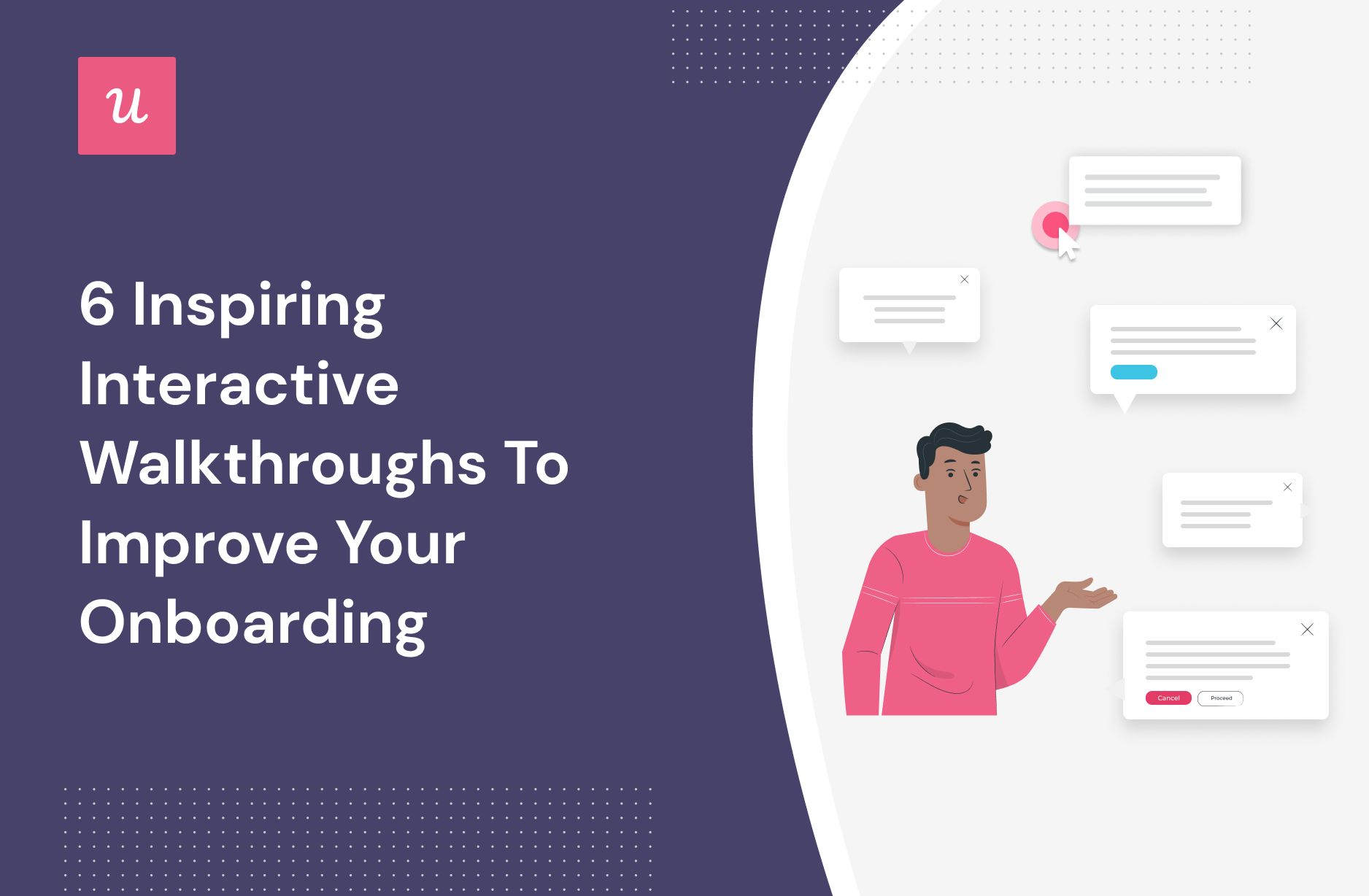This image features a rectangular advertisement or slide, longer than it is tall, potentially designed for an online platform or presentation. The left half of the image features a purplish or dark blue background with white lettering that reads, "six inspiring interactive walkthroughs to improve your onboarding." In the upper-left corner sits a lowercase letter "U" in white, enclosed within a pink or red square, followed by a pattern of white dots beneath the text.

On the right side, against a lighter or white background, a cartoon illustration of a young man of color with short, dark hair is depicted. The man wears a pink shirt with white stripes on the collar and across the middle. His left hand is raised, palm up, as though presenting five thought or speech bubbles above his head. These bubbles are index card-like illustrations with varied designs: one is white with a pink circle, another has blue at the bottom, and yet another combines red and white colors. Positioned as though emerging from the man's hand, the bubbles suggest different talking points or concepts, possibly related to the "interactive walkthroughs" mentioned in the text. The overall design emphasizes a modern, engaging visual meant to capture attention and convey information about improving onboarding experiences.